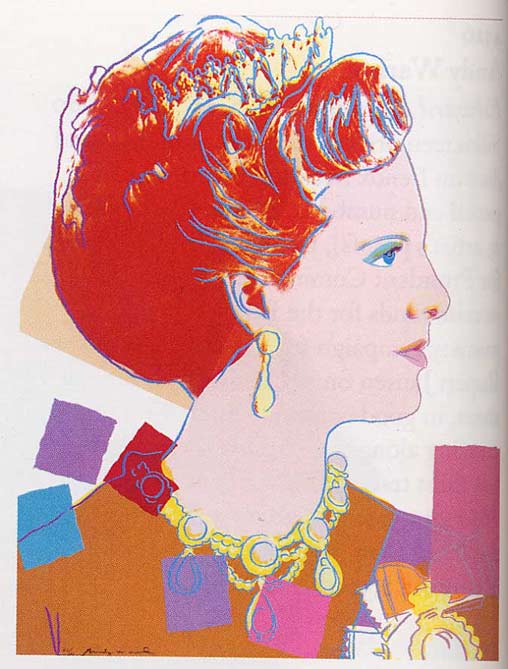This vibrant, museum-worthy work of pop art showcases a side profile of a striking woman with vivid, porcelain skin and intense blue eyes. Her short red hair is highlighted with streaks of yellow and blue and is adorned with a subtle whitish crown at the top. She has blue eyeliner and eyebrows that accentuate her expressive features, red-tinted nostrils, and pale pink lips. The woman wears large dangling golden earrings and a distinct golden necklace featuring evenly spaced balls. Her attire includes a brown shirt or dress with a purple strap across the right shoulder, adorned with a white flowery badge.

The background and her clothing are dotted with floating geometric shapes: blue, red, purple, pink, and orange squares add a dynamic, rhythmic visual element. Particularly, a red square is on her shoulder, a purple one is near her necklace, and strategically positioned around her neck area are squares in various hues, including blue, red, purple, pink, and dull pink. The surrounding wall features a dark, slightly brown backdrop contrasting with lighter shades, enhancing the artwork's depth and complexity.

This multicolored painting is postcard-sized and its intricate details and lively color palette give it a unique presence, marking it as a true piece of art fit for display in a distinguished gallery.